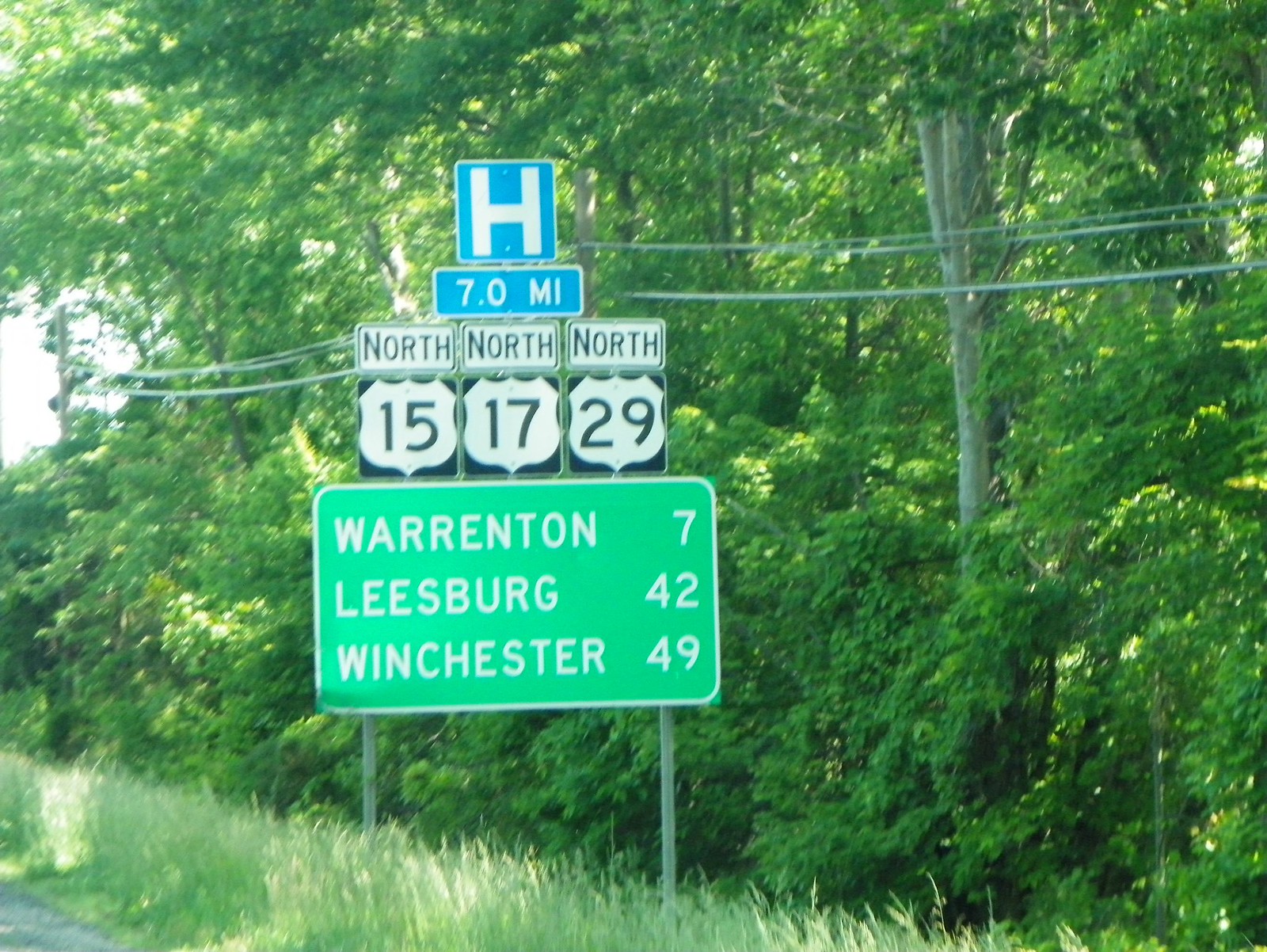This vibrant, scenic photograph captures a highway sign amidst a lush, verdant landscape, typical of a summer day. The sign, supported by two posts, features multiple panels. The bottom green sign displays in large white capitalized text: "Warrington 7," "Leesburg 42," and "Winchester 49." Above this are three white highway shields indicating "North 15," "North 17," and "North 29" in black letters. Topping the assembly is a square, blue hospital sign with a bold white 'H' and an accompanying rectangular sign below it that reads "7 miles," highlighting the distance to the nearest hospital. The backdrop reveals a dense array of lush green trees and some tall grasses with visible seed heads, supplemented by utility wires hanging behind the sign. Likely located in Virginia, given the mentioned cities and highway numbers, this scene epitomizes a summer drive in or near Warrington, Virginia.